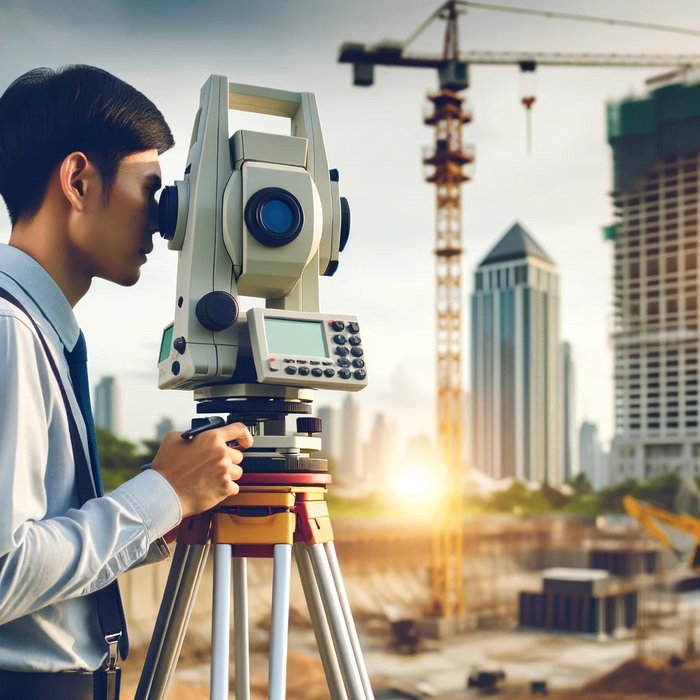In this AI-generated image, which has a realistic yet slightly cartoonish tone, a young Asian man with neatly groomed black hair and sideburns is seen from the waist up on the left side. He is wearing a light blue shirt, a black belt, and possibly blue tie and suspenders, although this detail is not entirely clear. His arms are bent at the elbows as he peers through a sophisticated piece of equipment, likely a survey instrument, which stands on four silver tripod legs. This device features multiple lenses, a digital display, a keyboard, and adjustable gears. In the background, set against a daytime sky, there are two buildings under construction. The building on the right is skeletal, revealing a framework of wood two-by-fours spanning two floors. Beside it to the left stands a slender black-and-white structure with a gray peaked roof. Overhead, a white and black crane extends from right to left. Further in the distance, skyscrapers and trees complete the urban construction scene.